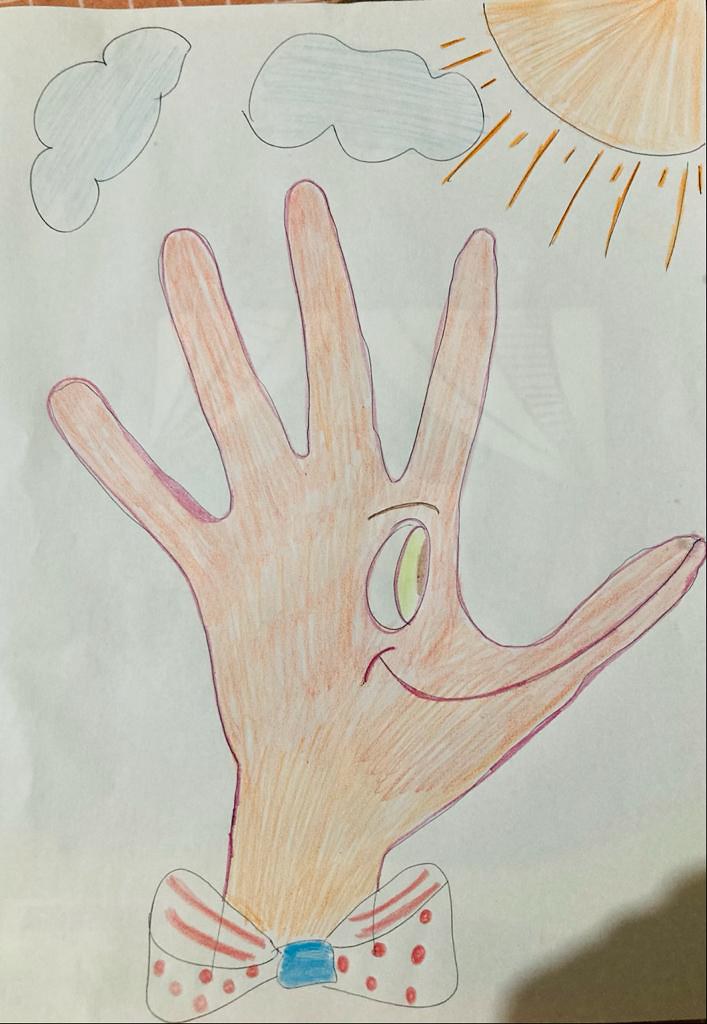A vibrant color pencil drawing on white paper showcases a creatively anthropomorphized hand. In the top right corner of the image, a peach-colored sun with radiating lines brightens the scene. Adjacent to this, on the top left, two simplistic cloud outlines in dark maroon pencil float in the sky. The central focus is the detailed outline of a hand traced in dark maroon or brown pencil and filled with peach tones. An intriguing feature is the singular eyeball, drawn within the hand, complete with a yellow pupil encircled by a dark brown ring. 

Extending from the thumb, a red or maroon line forms a whimsical smile, with a small dash line acting as the nose, giving the thumb a joyful expression. The wrist area is adorned with a charming bow tie, outlined in white with a light black edging, filled with red lines and tiny dots, and highlighted with a blue center square. The overall artistic vision transforms the hand tracing into a lively character, complete with a bow tie, suggesting a side profile of a smiling face.